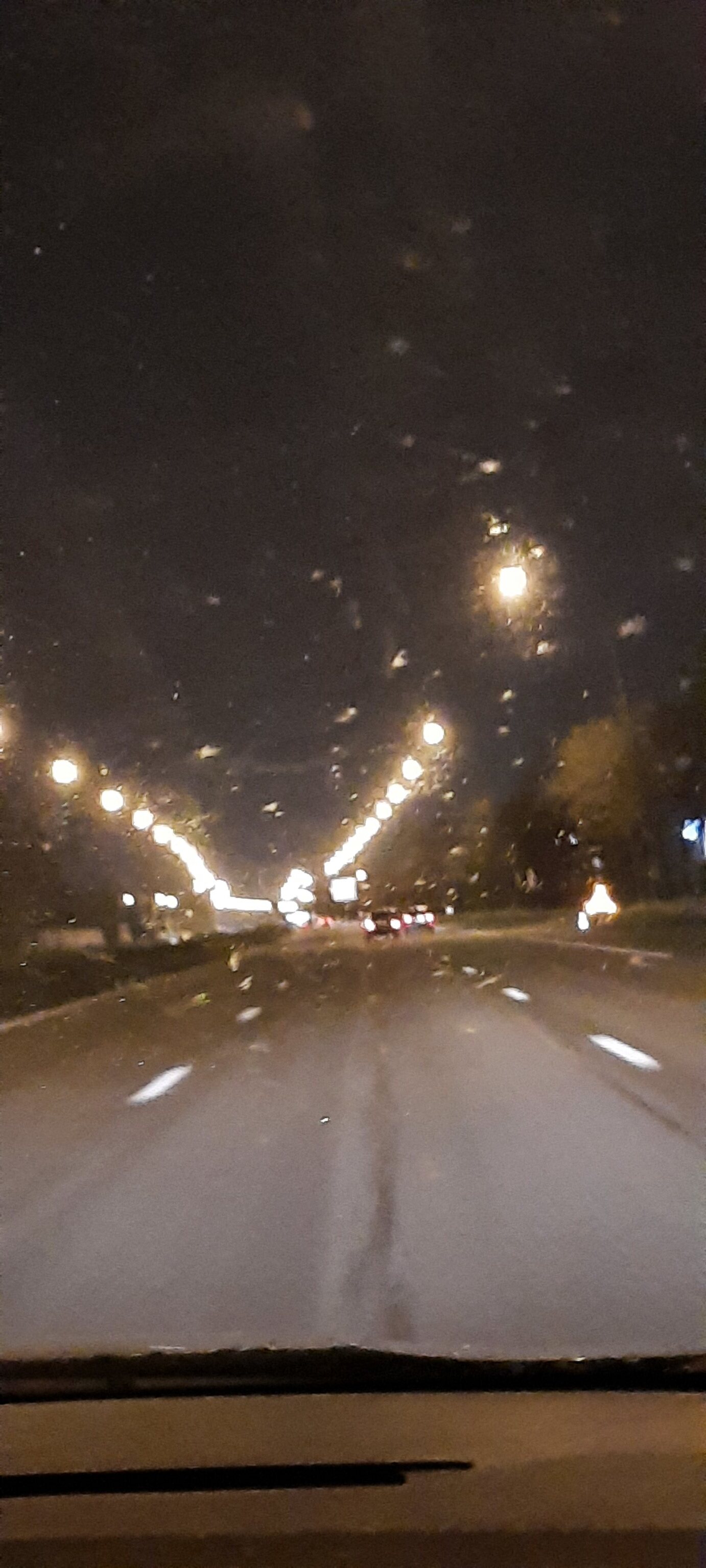A rainy night drive is captured in this image, with water droplets scattered across the windshield, reflecting the bright glow of streetlights. The scene is illuminated by both the streetlights overhead and lights from passing cars. The perspective is from the inside of the car, showing a part of the dashboard. Ahead, two vehicles are visible on the road. The street itself is a three-lane road marked by two rows of dashed lines. Trees line the side of the road, their shapes faintly visible in the dim light. A divider separates the lanes, indicating there is likely another street parallel on the other side. The sky above is pitch black, devoid of any stars or the moon, emphasizing the darkness of the night.